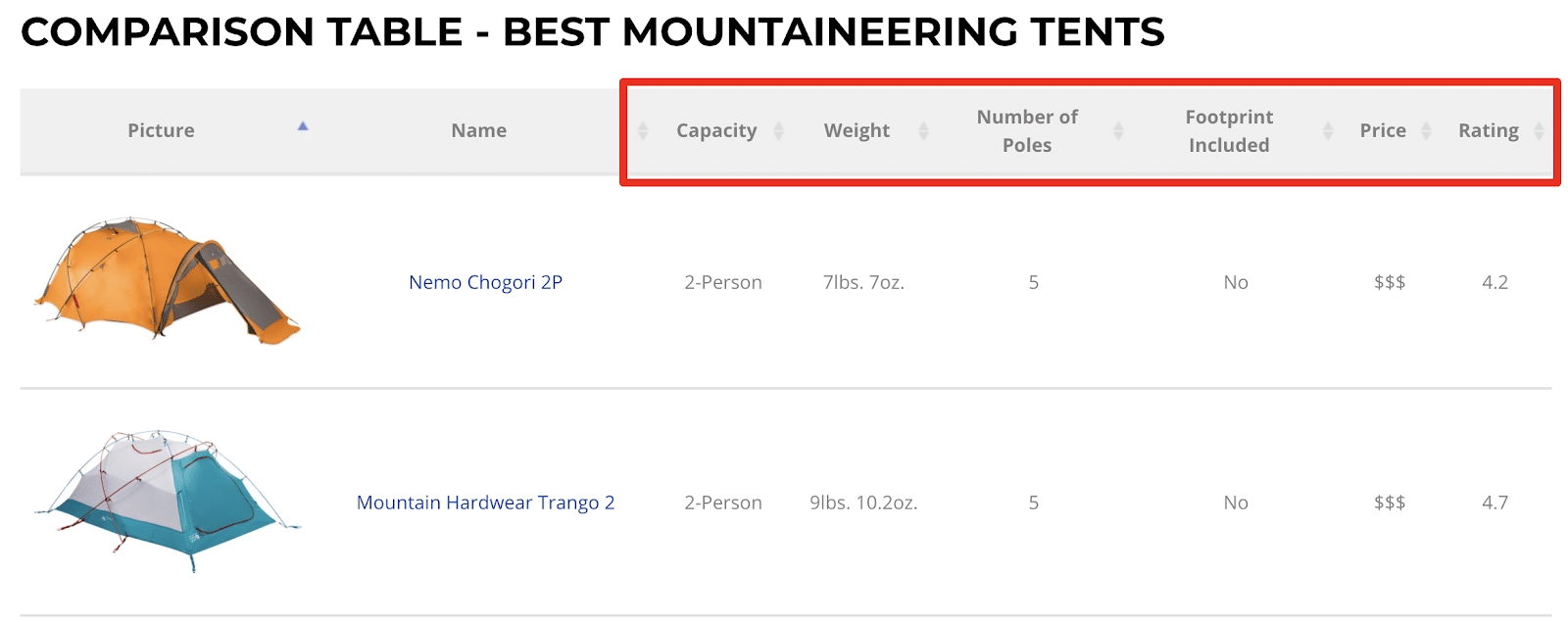**Detailed Comparison Table of Best Mountaineering Tents**

This educational image features a comprehensive comparison table of the best mountaineering tents. Dominating the top part of the table, the title "BEST MOUNTAINEERING TENTS" is prominently displayed in large black capital letters. Immediately beneath the title, a gray bar spans across the image, categorizing the table columns: Picture, Name, Capacity, Weight, Number of Poles, Footprint Included, Price, and Rating. 

An eye-catching red border encapsulates the columns from Capacity to Rating, emphasizing these specific details. 

Towards the left side of the table, two tents are showcased in their fully assembled forms:

1. **Nemo Chogorinp 2P**:
   - **Appearance**: Orange tent
   - **Name**: Nemo Chogorinp 2P 
   - **Capacity**: 2 persons
   - **Weight**: 7 pounds, 7 ounces
   - **Number of Poles**: 5
   - **Footprint Included**: No
   - **Price**: $$$ 
   - **Rating**: 4.2

2. **Mountaineer Hardware Trango 2**:
   - **Appearance**: Teal green and white tent
   - **Name**: Mountaineer Hardware Trango 2
   - **Capacity**: 2 persons
   - **Weight**: 9 pounds, 10.2 ounces
   - **Number of Poles**: 5
   - **Footprint Included**: No
   - **Price**: $$$
   - **Rating**: 4.7

The background of the image is white, accentuated with various colors such as black, gray, red, yellow, brown, blue, and teal, contributing to the visual appeal and informational clarity of the table.